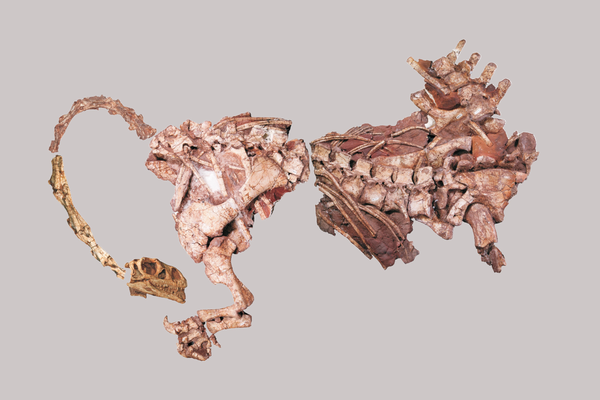The photograph displays a skeletal structure of what appears to be a small creature, set against a light lilac background. The image is rectangular in shape and shows the skeleton in varying shades of white, brown, and tan. 

Prominently featured is an arched section that resembles a tail, leading to a small rectangular segment below it. Attached to this central piece is a portion of the pelvis or hip area, from which a leg extends downward, complete with foot bones. This structure suggests the hind part of the creature. 

Moving upwards, there is a visible but somewhat disjointed spinal column which is separated from the front section of the skeleton. Near this area, remnants of a front leg can be seen, though it appears broken and incomplete. The right side of the image shows a relatively larger chest cavity, and above it, there is an indistinct shape that might be part of the head, though its features are not clearly discernible.

Overall, the photograph presents a partial and possibly fragmented skeleton, providing intriguing details that spark curiosity about the creature’s identity and the narrative behind its preservation.